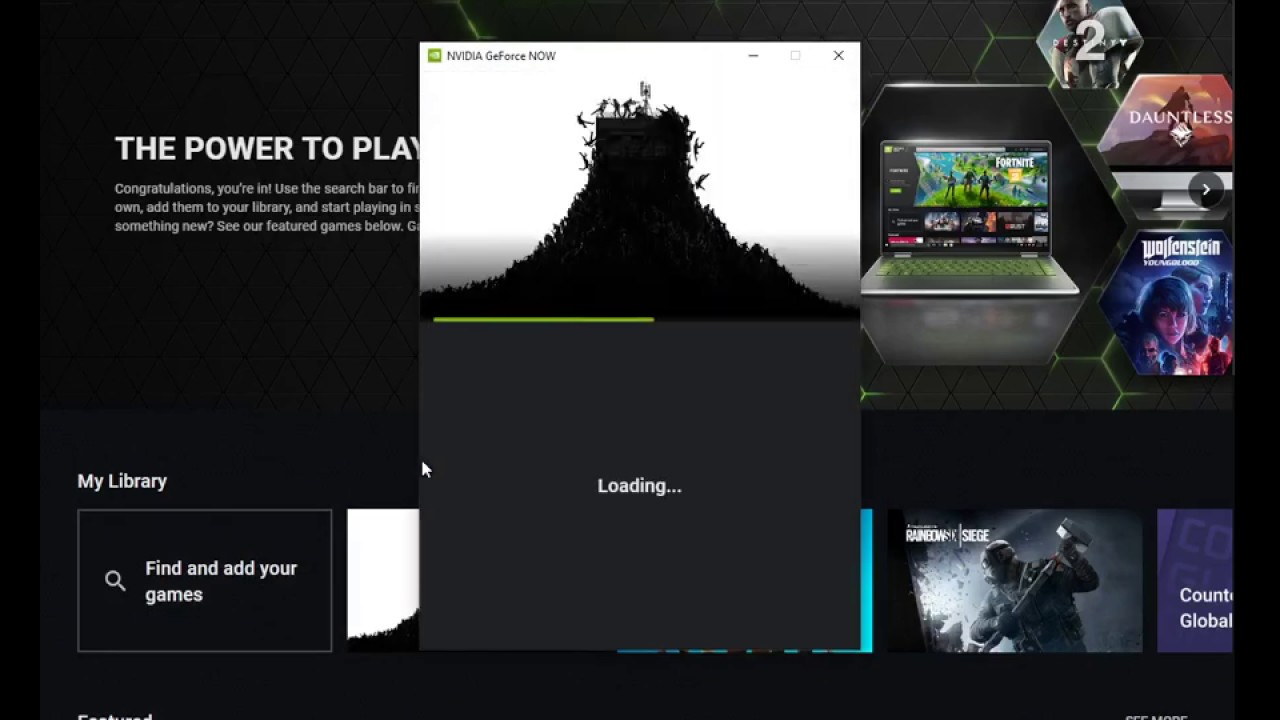In the image, we see a screenshot of a web page featuring the interface of NVIDIA GeForce Now, set against what appears to be a Windows operating system. The main focus is a vertical rectangular overlay in the center of the screen. The top half of this rectangle has a white background, dominated by a striking black silhouette that resembles a volcano. Tiny human figures are depicted scaling the "volcano," adding a sense of dynamic activity to the silhouette.

Beneath this graphical element, a green loading bar stretches halfway across the screen, indicating that something is in the process of loading. Directly below the loading bar, there's a gray square section. At the center of this square section, the words "Loading..." are prominently displayed in white text.

Surrounding this central vertical rectangle, we observe the broader NVIDIA GeForce Now interface. On the left side of the screen, partially obscured by the overlay, is a section with the words "The power to play." Further down on the bottom left, the phrase "My Library" is visible in white text set against a black background. Below this, there is another square with a thin gray border, containing the text "Find and add your games" in white, accompanied by a magnifying glass icon on its left side. Towards the middle of this gray-outlined square, several other gray squares are arranged horizontally, showcasing various games likely present in the user's library.

The detailed layering and design elements highlight the interactive and user-centric experience of the NVIDIA GeForce Now interface, emphasizing both functionality and aesthetics.